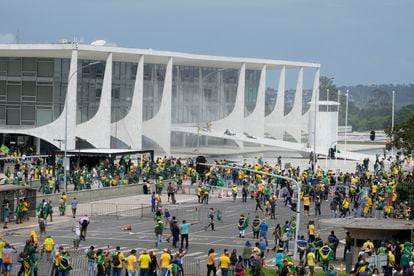The image depicts a bustling city street teeming with people, centered around a large, modern white building with distinctive and oddly shaped columns. The building, likely an architectural focal point, stretches from the left to the right in the background. Below it lies a gray asphalt road filled with crowds of people, some of whom are dressed in yellow shirts, suggesting they may belong to a group participating in an event, possibly a protest or a marathon. The scene is set outdoors, with a clear blue sky overhead. There are also green trees visible in the background on the right side, and a silver pole is prominently positioned in the foreground, adding to the dynamic urban atmosphere. No text or signage is visible in the image, leaving the specific location indeterminate. The overall setting conveys the lively and energetic ambiance of a city street during a significant public gathering.